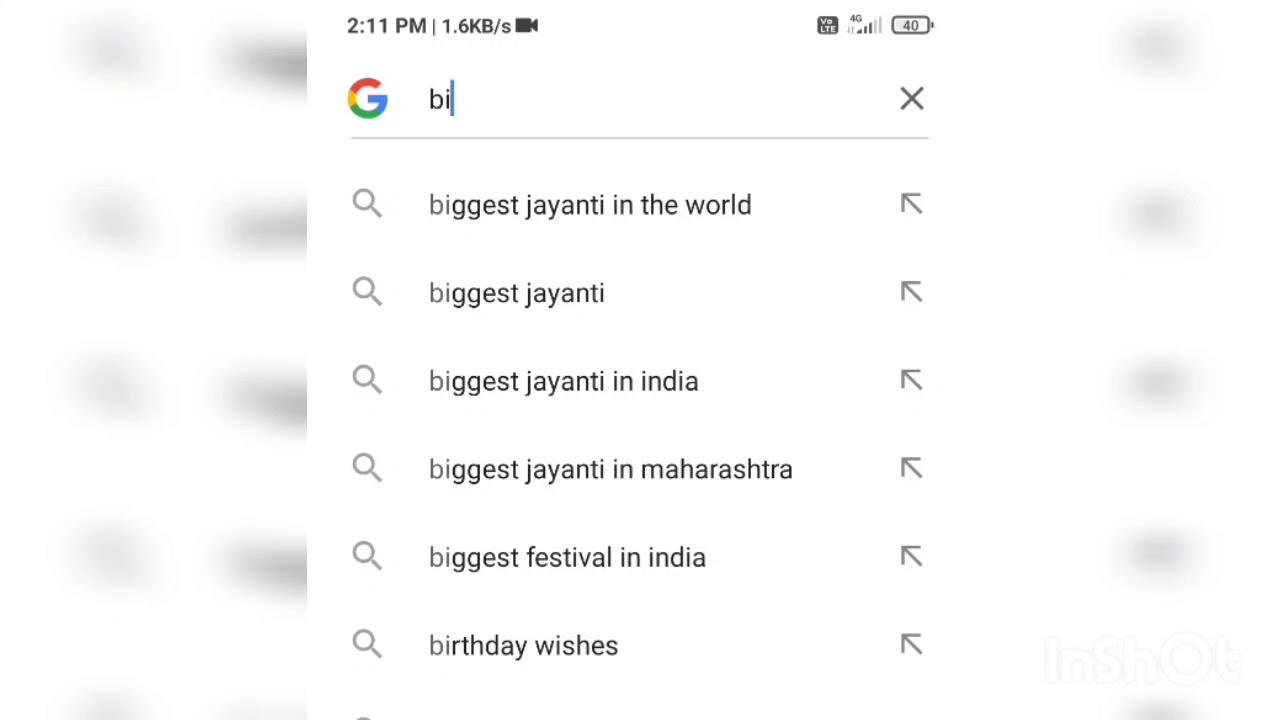The image captures a section of a Google search page displayed on a mobile phone. This is evident from the various status icons visible at the top right corner of the screen, including a battery indicator showing 40% charge, a 4G network signal represented by progressively taller vertical bars, and a small black square presumably displaying the phone carrier's name. Additionally, the left side of the status bar shows the current time, 2:11 PM, alongside a data speed rate of 1.6 kilobytes per second, and a camera icon.

The focal point of the image is the Google search interface itself. At the top, the iconic multicolored Google 'G' logo is prominently displayed, featuring a capital letter 'G' with segments in red, orange, yellow, green, and two shades of blue. Below the logo, a user has begun typing the letters "B I" into the search bar. Consequently, Google has generated several autocomplete suggestions tailored to the user's potential queries. The suggestions listed are:

1. "Biggest Jayanti in the world"
2. "Biggest Jayanti"
3. "Biggest Jayanti in India"
4. "Biggest Jayanti in Maharashtra"
5. "Biggest festival in India"
6. "Birthday wishes"

Each of these suggestions is accompanied by a magnifying glass icon on the left, indicating they are search queries, and an arrow pointing upwards towards the top left on the right, suggesting these are clickable links that will direct the user to their respective search results.